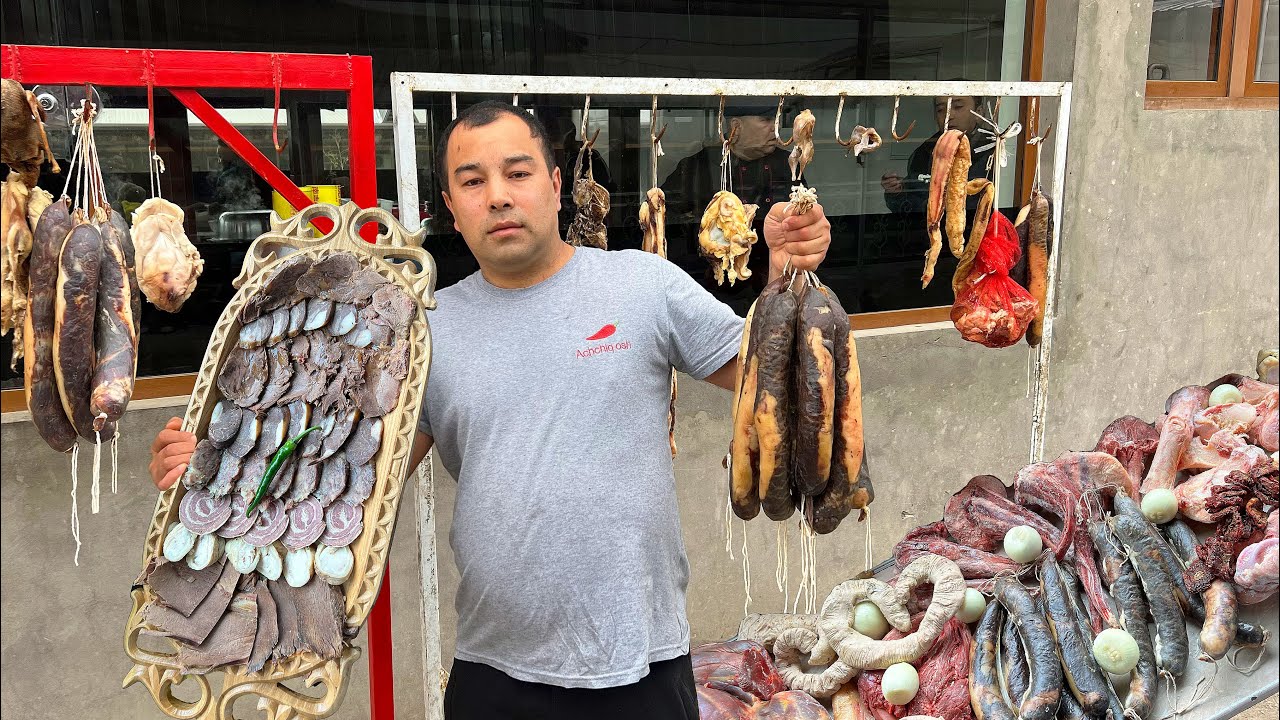The photograph captures an Asian man standing in what appears to be a butcher shop or a meat market. He is wearing a gray t-shirt with a small red chili logo on the chest and black pants. In one hand, he holds a white basket filled with various cuts of meat, while in the other hand, he raises a bunch of large sausages that are black and yellow. Behind him, there are two racks: a red hanging rack and a white rack, both adorned with raw meats and sausages dangling from metal hooks. To his side, or slightly behind him, is a table laden with an assortment of meat that appears unappetizing and raw. The setting is brightly lit, suggesting it was taken outdoors during the daytime, adding to the clarity and detail of the image.